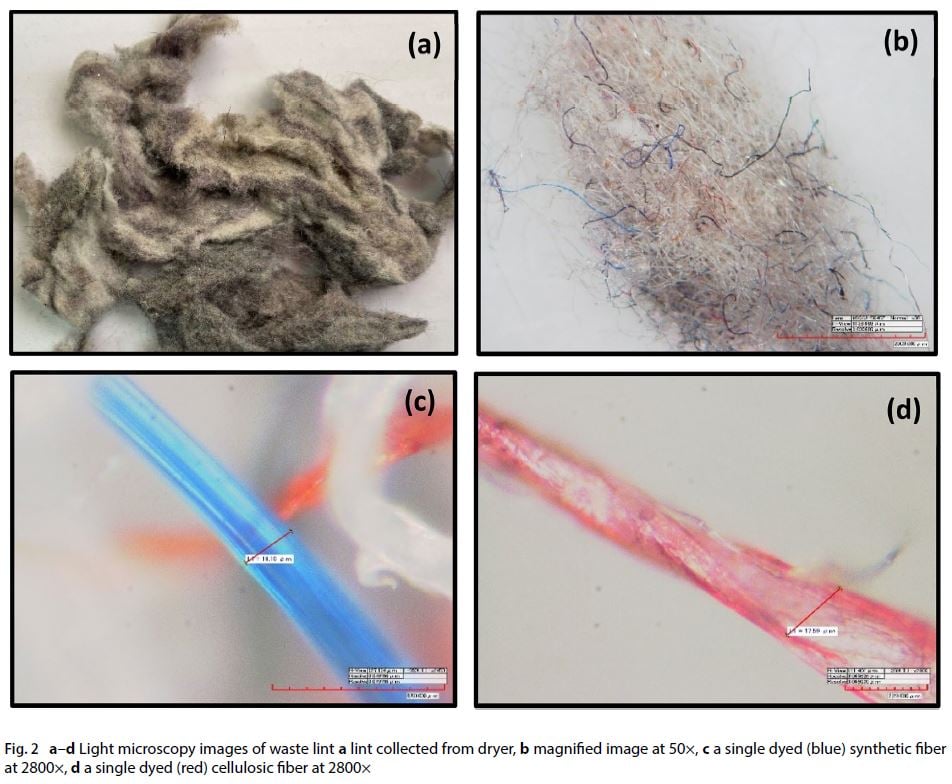The image is a mosaic of four equally-sized photographs labeled A, B, C, and D in the top right corners, respectively. Each photo provides a progressive zoom into the material being analyzed. 

Photo A, positioned at the top left, depicts a large mound of dark-colored dryer lint. In the adjacent Photo B, a closer look at a portion of this dryer lint reveals an intricate mix of gray and blue fibers, magnified by a factor between 5 and 50 times. Moving to the bottom left, Photo C presents a highly magnified view (2,800x) of a single blue synthetic fiber extracted from the lint. Finally, Photo D in the bottom right displays another fiber at the same magnification (2,800x) — this time a single red cellulosic fiber. Each image is accompanied by detailed notations indicating the specific materials and magnifications used in the analysis.